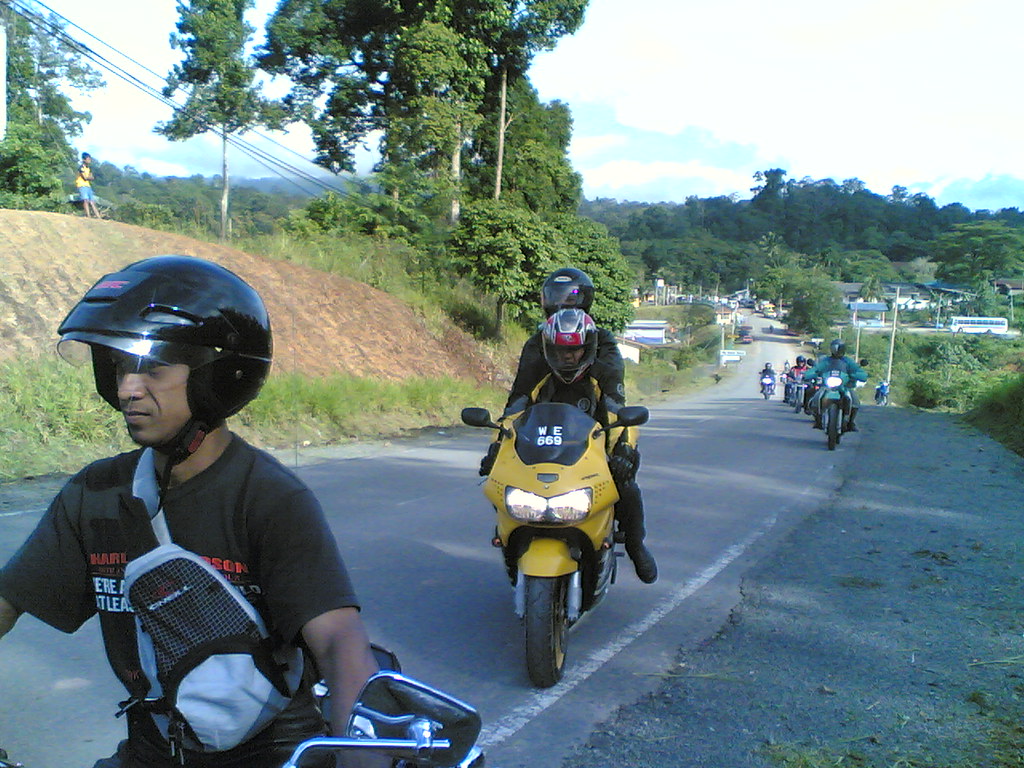The photograph captures a vibrant scene of multiple motorcyclists riding uphill on a gray asphalt road, clearly marked with a dotted white center line and solid white edge lines. The road, flanked on both sides by lush green vegetation, stretches far into the distance where a small town with multiple buildings, a bus, and more cars is visible. On the left side of the image, there's a steep slope with brown patches, topped with trees, telephone poles, and wires. The right side features a gravel shoulder area with more dense vegetation. The bright light blue sky, dotted with white and gray clouds, provides a scenic backdrop. 

In the foreground, the leading motorcyclist, positioned on the front left, is wearing a black helmet and black t-shirt. Following him is a yellow motorcycle carrying two riders dressed in black. Behind them, a teal motorcycle is visible, followed by a diverse group of riders on motorcycles of various colors including green, blue, red, and black, though these are somewhat harder to distinguish in the distance. The overall perspective gives a sense of movement and adventure as the road inclines and curves towards the horizon.